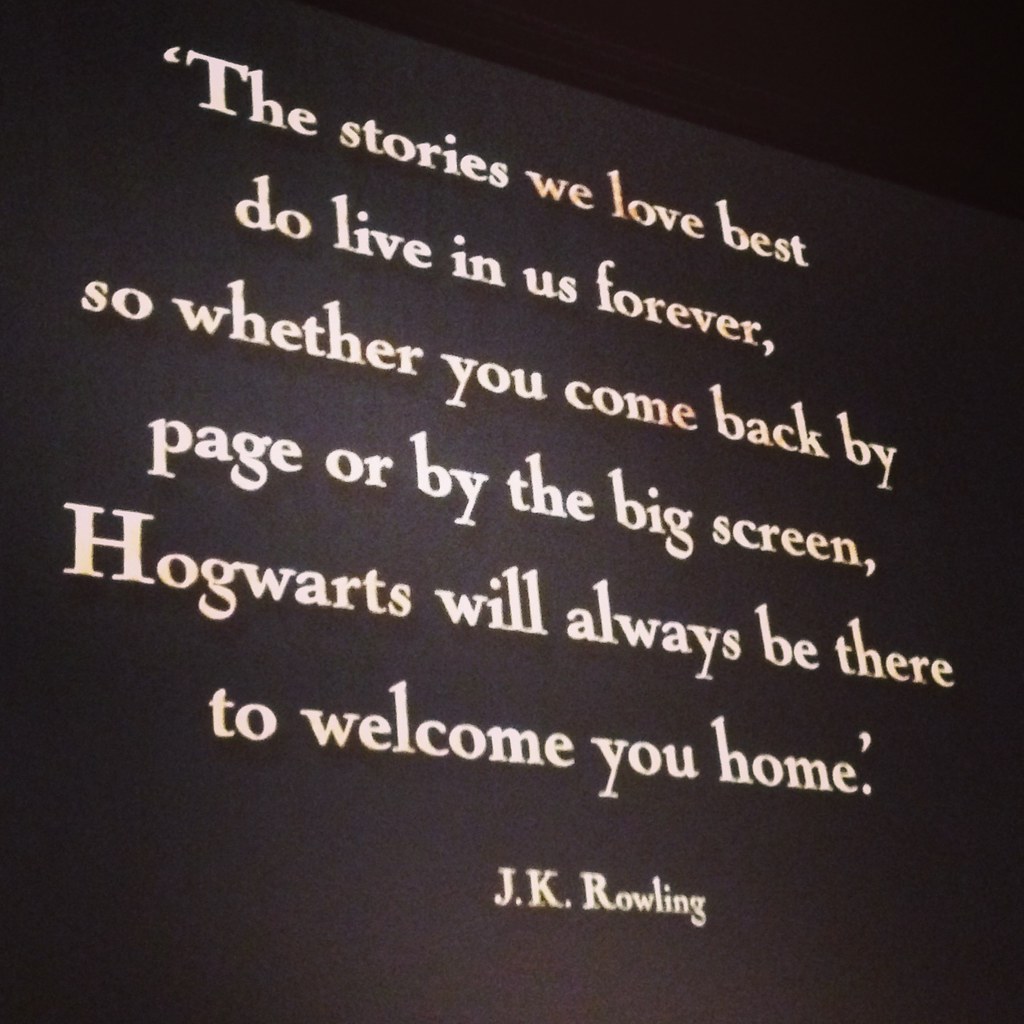The image depicts a slightly grainy, somewhat blurry projection on a primarily black screen, possibly in a movie theater or on a large display in a dark setting. The text is prominently displayed in big, off-white letters and reads: "The stories we love best do live in us forever, so whether you come back by page or by the big screen, Hogwarts will always be there to welcome you home." Below this quote, in smaller letters, is the name "J.K. Rowling." The text appears to be slightly angled, suggesting the photo was taken from the left side. Various shades of black in the background further hint at the screen's surface texture.